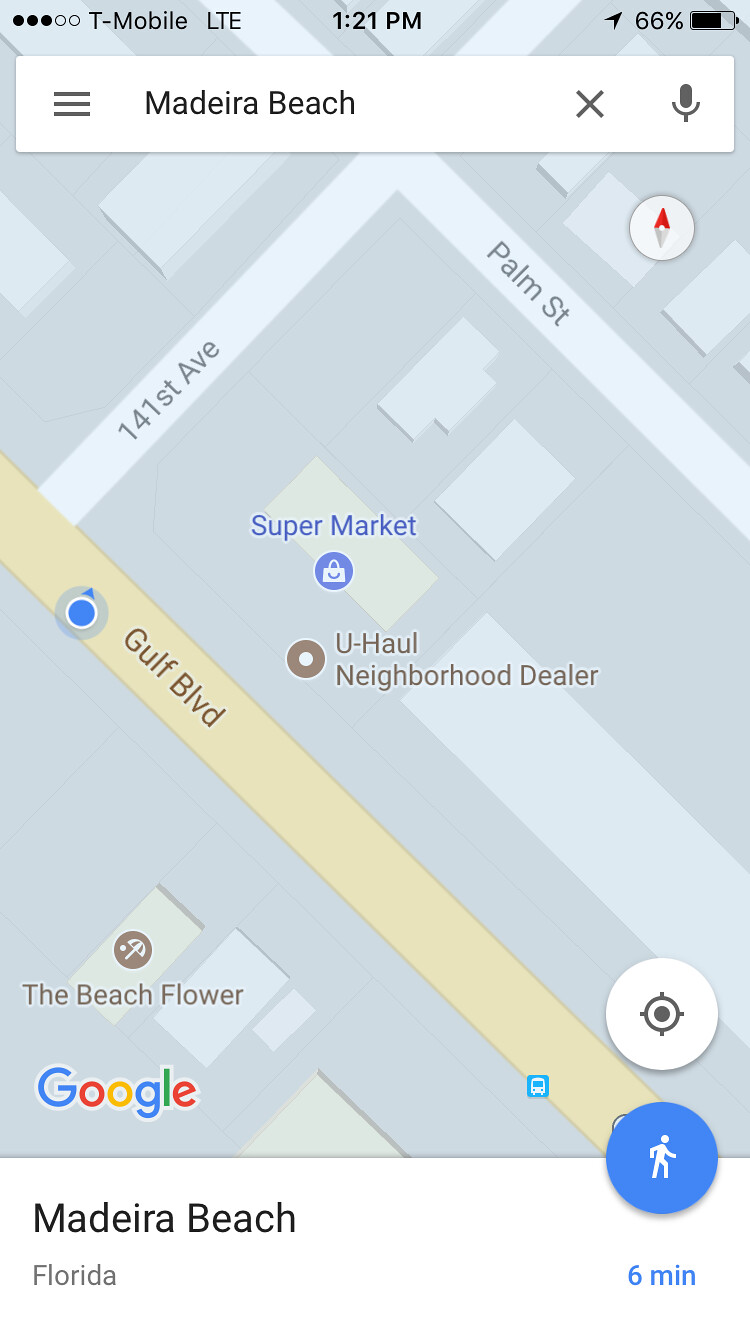The image appears to be a screenshot from a smartphone displaying a section of a Google Maps interface. At the top of the screen, the phone's status indicators show a T-Mobile LTE connection with moderate signal strength, represented by five circles with three filled in and two hollow. The battery level is at 66%, and an icon indicates that location services are active.

The map is highly zoomed in on an area in Madeira Beach, Florida, specifically focusing on a U-Haul Neighborhood Dealer. Also noticeable nearby is a building labeled as a supermarket. Prominently featured on the map is Gulf Boulevard, a main road likely named due to its proximity to the Gulf of Mexico. In the lower-left section of the map, there's a label for "The Beach Flower," which could be another point of interest or business.

The bottom-left corner of the image features the Google Maps icon, and a blue circle with a walking person indicates that the user has selected walking directions for their journey. The planned route will take approximately six minutes. A blue location marker on the map shows the user's current position, which appears to be heading northeast towards 141st Avenue, where it intersects with Palm Street.

Currently, the map view does not show the step-by-step directions, but it is clear that the person is on their way to their destination.